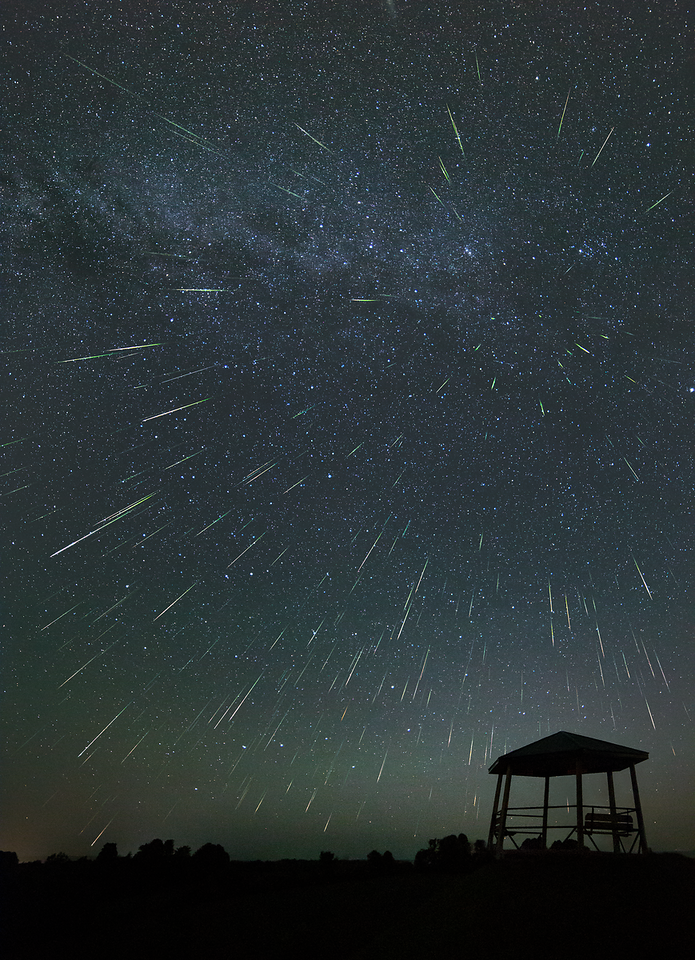Underneath an expansive night sky, filled with countless tiny white dots that resemble stars, a multitude of thin, vibrant streaks of yellow and white—accompanied by occasional red and blue sparks—shoot across the sky in various directions, mostly downwards. This sky, gradient from dark black to a grayish hue due to the density of stars, appears almost otherworldly, as if viewed from outer space. Towards the upper center-right area, the shooting stars converge and spread outwards. A noticeable white cloudy patch further enhances the celestial display. 

Below this celestial spectacle, the dark silhouette of the earth's top edge is visible. Nestled in the bottom right corner of the image, an observatory with a flat roof supported by posts stands in shadow, rendering it almost entirely black. A bench lies beneath this sheltered area. The horizon line features intermittent bushes, though the terrain itself is primarily level, contrasting with the star-laden sky above.